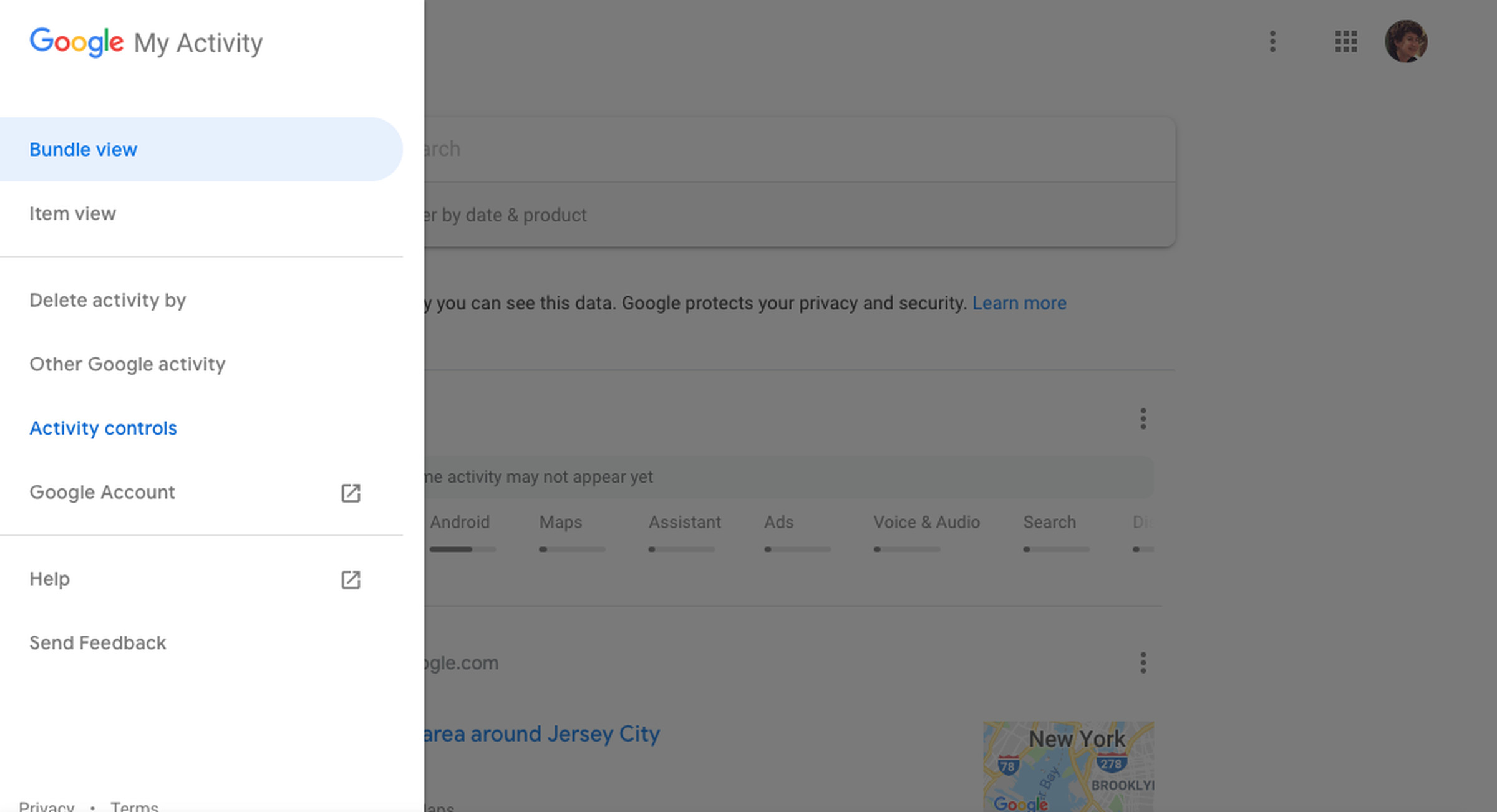The image in question is a screenshot captured from a computer screen, distinguished by its widescreen format. The main content appears to be a Google settings page. On the left side of the image, there is a white-background section that resembles a side menu titled "My Activity." This menu lists several options such as "View Bundle," "Item View," "Delete Activity," "My Other Google Activity," "Activity Controls," "Google Account," "Help," and "Send Feedback," arranged in a vertical list, almost resembling a pop-up window.

On the right side of the screenshot, the Google settings interface is visible but appears dim and shadowed. In the top right corner, the user's Google account profile picture is displayed. The page also contains various features, including what looks like a small map of New York, along with several security settings options.